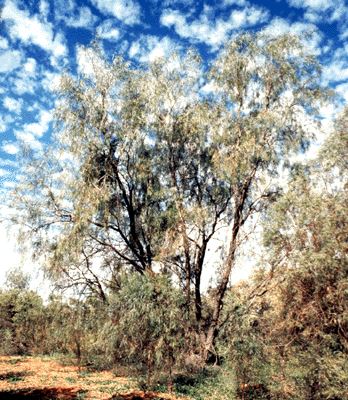The photograph depicts a natural scene dominated by a tall, central tree with multiple branches emerging near its base, giving the impression of several trees fused into one. The tree and surrounding shrubs appear somewhat dried with a mix of green and brown shades, hinting at sparse foliage. At the bottom left of the image, there is a light brown ground with an orange hue. The green shrubs and short brush-like trees are scattered across the foreground, including the bottom right, adding to the texture of the scene. Above, the sky is a striking deep blue, adorned with scattered white clouds that become bright white near the center. This rich blue sky with puffy clouds provides a vivid backdrop to the otherwise earthy and subdued tones of the trees and shrubbery below.